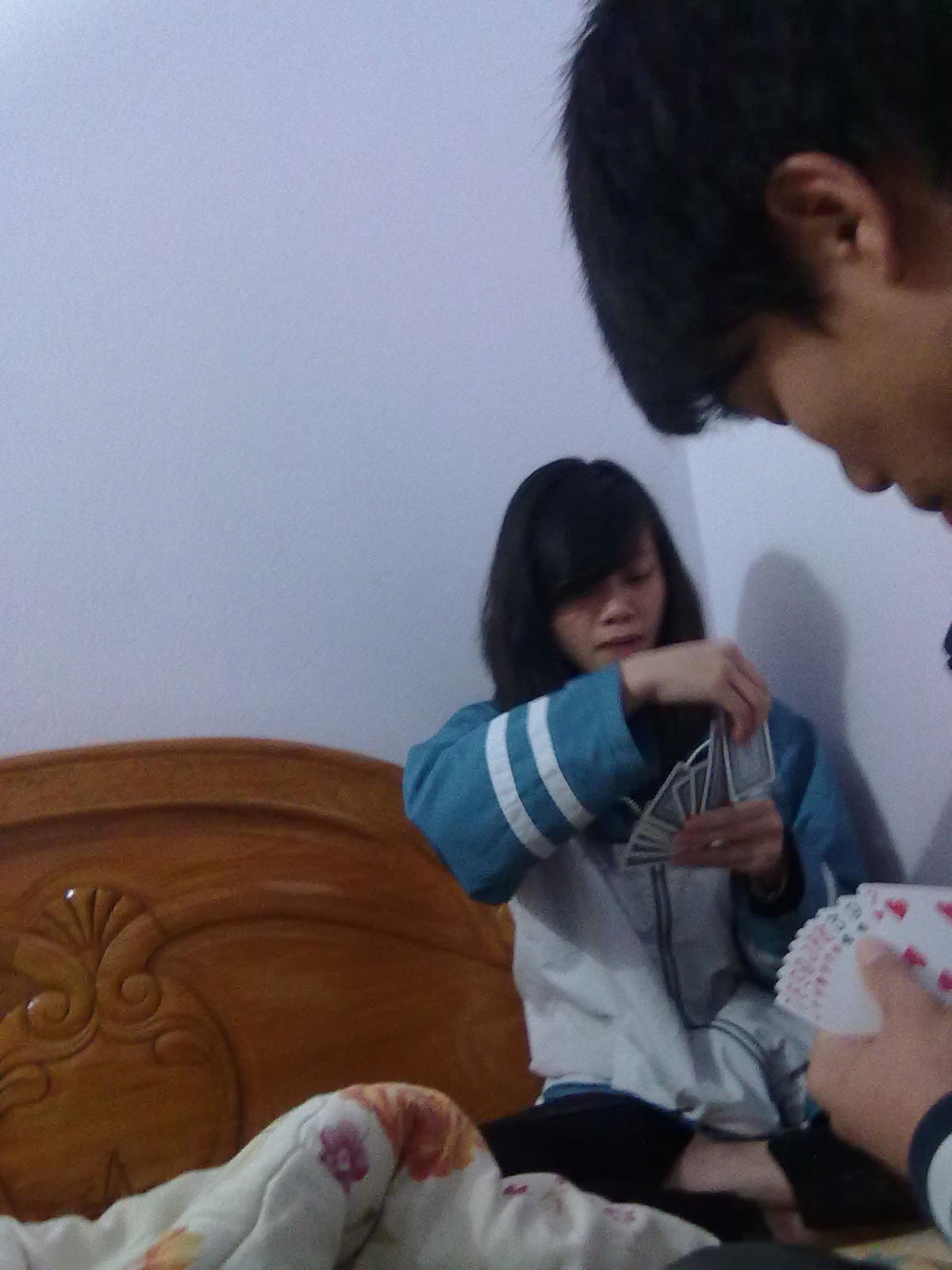In a cozy bedroom with light lilac walls, two people are seated on a bed, engaged in an intense game of cards. The ornately detailed dark wooden headboard provides a rich contrast to the room's soothing color scheme. A girl sits closest to the headboard, her right side adjacent to the wall, casting a soft shadow. She has dark hair with bangs and wears a white baggy shirt with blue and white sleeves, sitting in a crisscross position. Holding a full deck of cards in one hand, she appears ready to pick a card from the deck with her other hand. Next to her is a man, his face partially visible, focused intently on his own hand of cards. He has dark hair and prominent features. Spread across the bed is a white quilt adorned with vibrant flowers in shades of orange, pink, and yellow, adding a touch of warmth and charm to the scene.